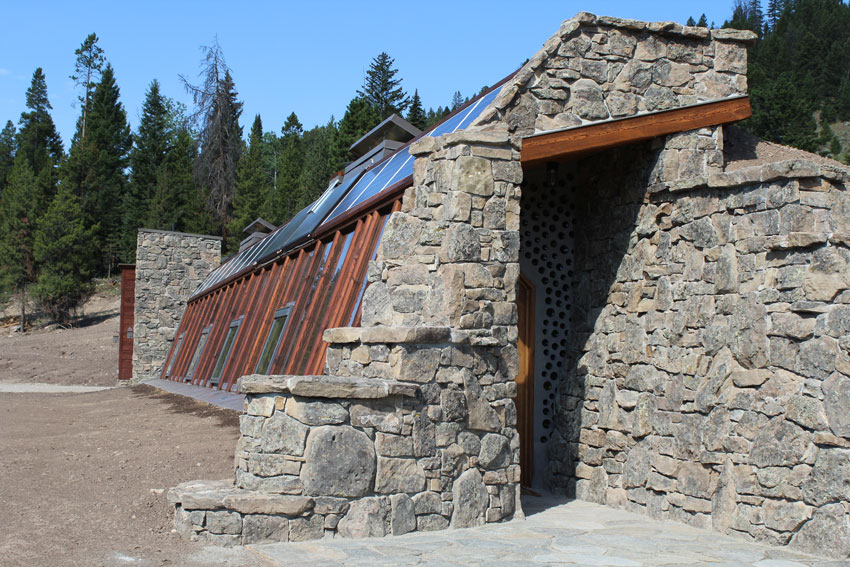This photograph showcases a rustic, elongated stone building nestled in a mountainous, evergreen setting under a vivid blue sky. The building, primarily composed of gray, possibly limestone stones of various shapes and sizes, features accents of brown, particularly noticeable in the wooden supports and eaves. Atop the structure, a distinctive roof integrates both solar panels and glass segments. The front entrance, slightly off to the right in the image, is adorned with decorations resembling dots on a white surface, and is flanked by stone pillars. Multiple windows are visible under the roof's slope and near the solar panels, while a stone chimney and additional wooden posts add to the architectural detail. The setting suggests it could be a visitor center or historic building, possibly located in a national park or a campsite, surrounded by dusty, grayish dirt paths and a backdrop of dense evergreen trees.